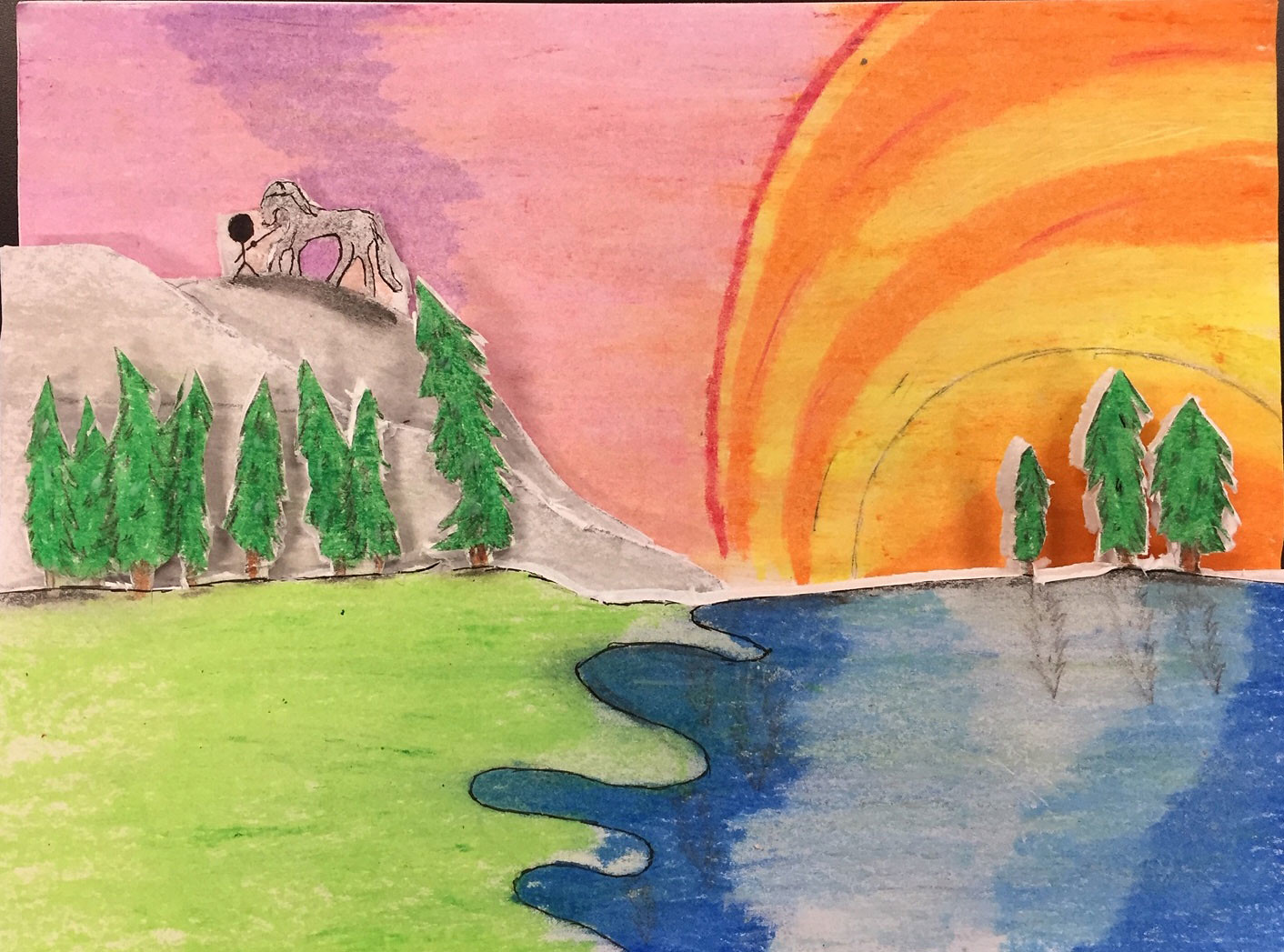The image depicts a vibrant, three-dimensional artwork that combines elements of traditional drawing with digital enhancements. The scene features a dynamic natural landscape with a diverse color palette. On the bottom left, lush green grass leads up to layered, green pine trees with brown trunks, reminiscent of Christmas trees. In the center, a towering grayish-brown mountain-like rock formation is partially obscured by these trees. Atop the rock, a stick figure dressed in black is seen holding a stick towards the neck of a grayish-brown horse. The right side of the image showcases a serene blue body of water, meeting the grass on the left. Above the water, a brilliant sunset of orange and yellow hues lights up the sky, transitioning to a pinkish-purple backdrop behind the mountain. The sun’s reflection casts a pale blue shimmer across the water, enhancing the tranquil atmosphere. The entire composition combines to create a vivid, nature-inspired artwork that feels both hand-crafted and digitally rendered.